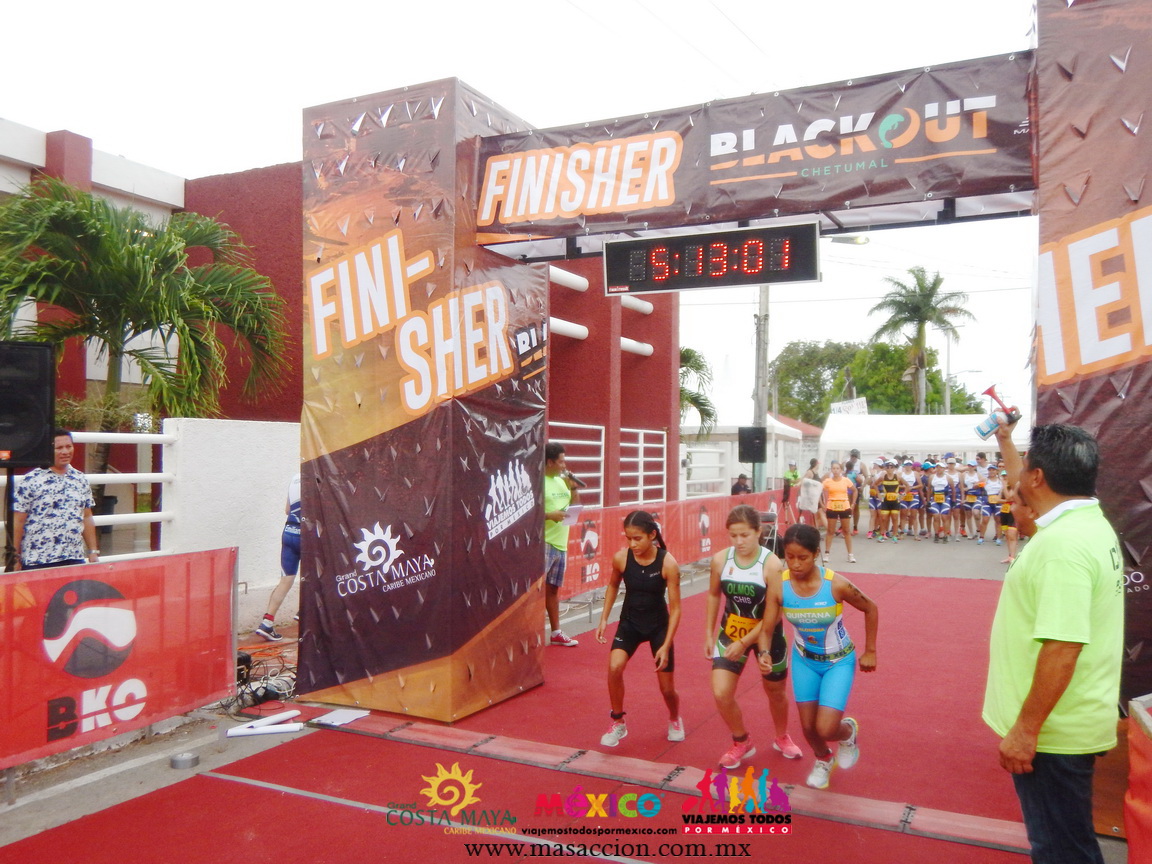The image captures the starting line of a children's relay race in Chetumal, Mexico, with prominent pillars displaying "Finisher" and "Blackout." Three young girls, approximately 12 to 13 years old, are at the forefront, ready to start running. The girl on the left has black hair in a ponytail, wearing a black Nike running jersey, black shorts, and white running shoes. The middle girl has brown hair in a ponytail, donning a white, black, and green running suit with pink shoes. To the right, the third girl, with black hair in a ponytail, wears a light blue, yellow, and purple running suit and white tennis shoes. A man in a green shirt stands to the side holding an air horn, signaling the start of the race. A group of runners is seen behind them, waiting for their turn. The clock in the background shows a time of 5 hours, 13 minutes, and 1 second. The event details can be found at www.machione.com.mx.